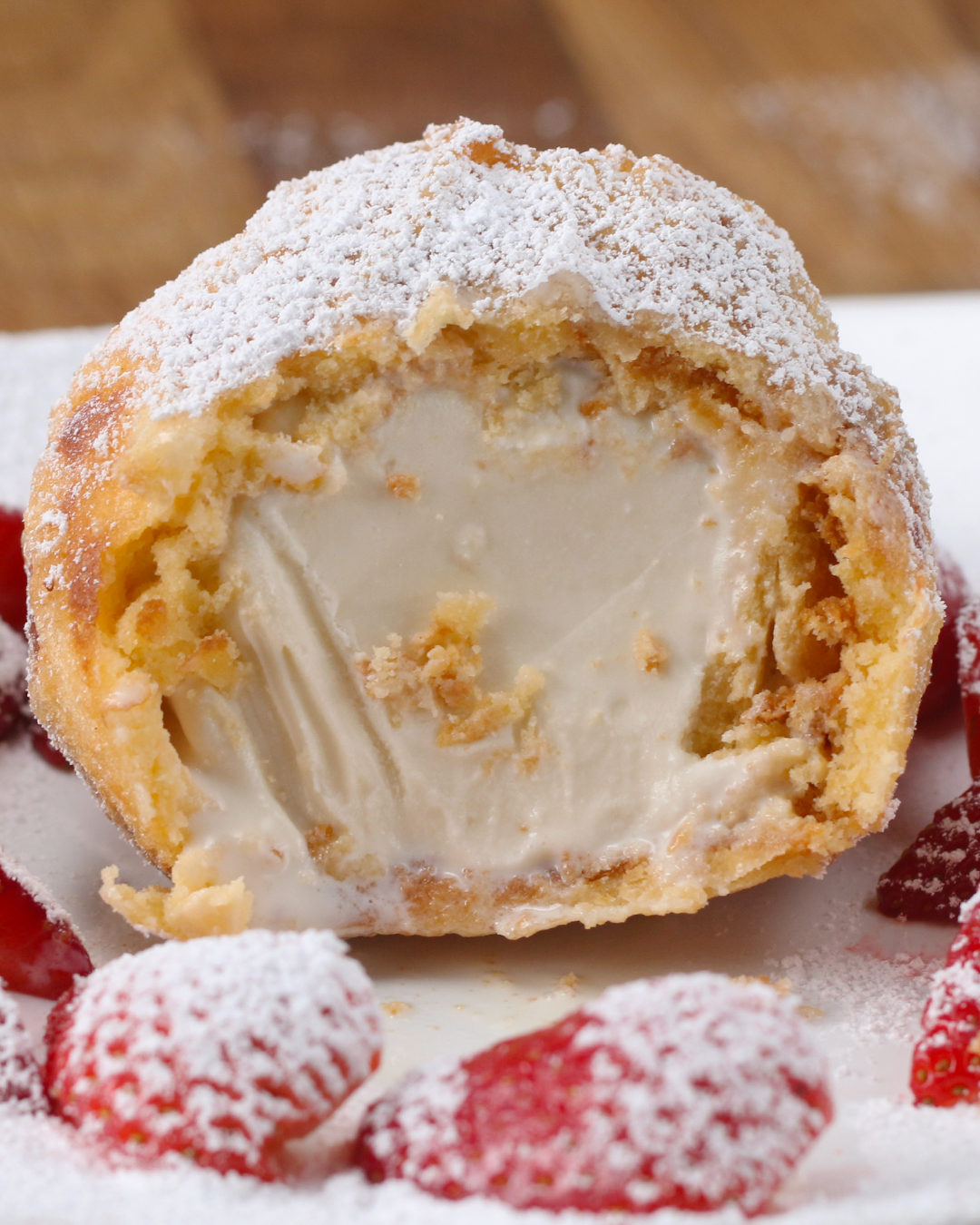This close-up photograph captures a round, tan pastry with a crusty exterior, dusted generously with powdered sugar. The front of the pastry is sliced open to reveal a rich, white cream filling, reminiscent of cream cheese or vanilla frosting. Surrounding the pastry, plump, sliced strawberries, also sprinkled with powdered sugar, rest on a pristine white plate. The background subtly showcases a wooden floor, out of focus to ensure the decadent dessert remains the focal point. The harmonious blend of the golden-brown crust, the creamy interior, and the vibrant red berries enhances the mouth-watering appeal of this delightful pastry, making it look irresistibly delicious.